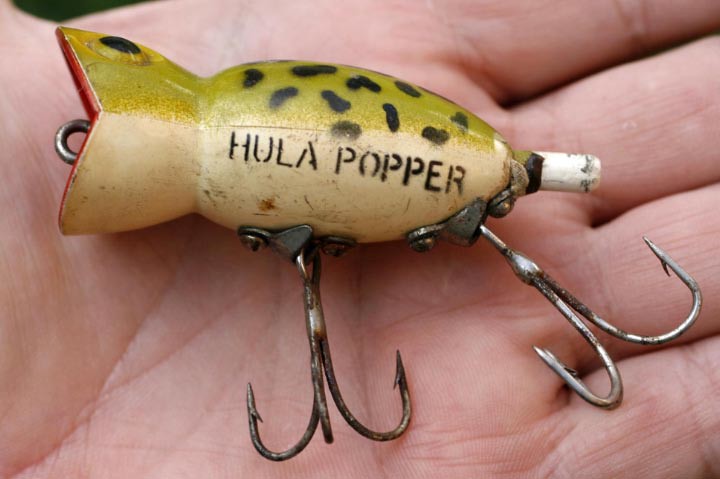A close-up image captures a fishing lure designed to resemble a small fish or frog, laying in the palm of a Caucasian person's left hand. The lure, which prominently features the brand name "Hula Popper" in black print, has a dual-tone color scheme: its top half is a bright green adorned with small black specks, while its bottom half is a yellowish off-white. The lure's mouth, open wide on the left side and displaying a dark pink or red interior, has a silver ring for attaching the fishing line. The front end of the lure also depicts a round, fish-like eye on the top left. Extending from the back end is a rounded white tail. The underside of the lure bristles with two treble hooks; the front hook is particularly rusty and dirty, with three sharp prongs, while the rear hook, less corroded, also sports three prongs. The image's close-up nature focuses solely on the lure and the palm, barely showing the hand’s fingers and lines.